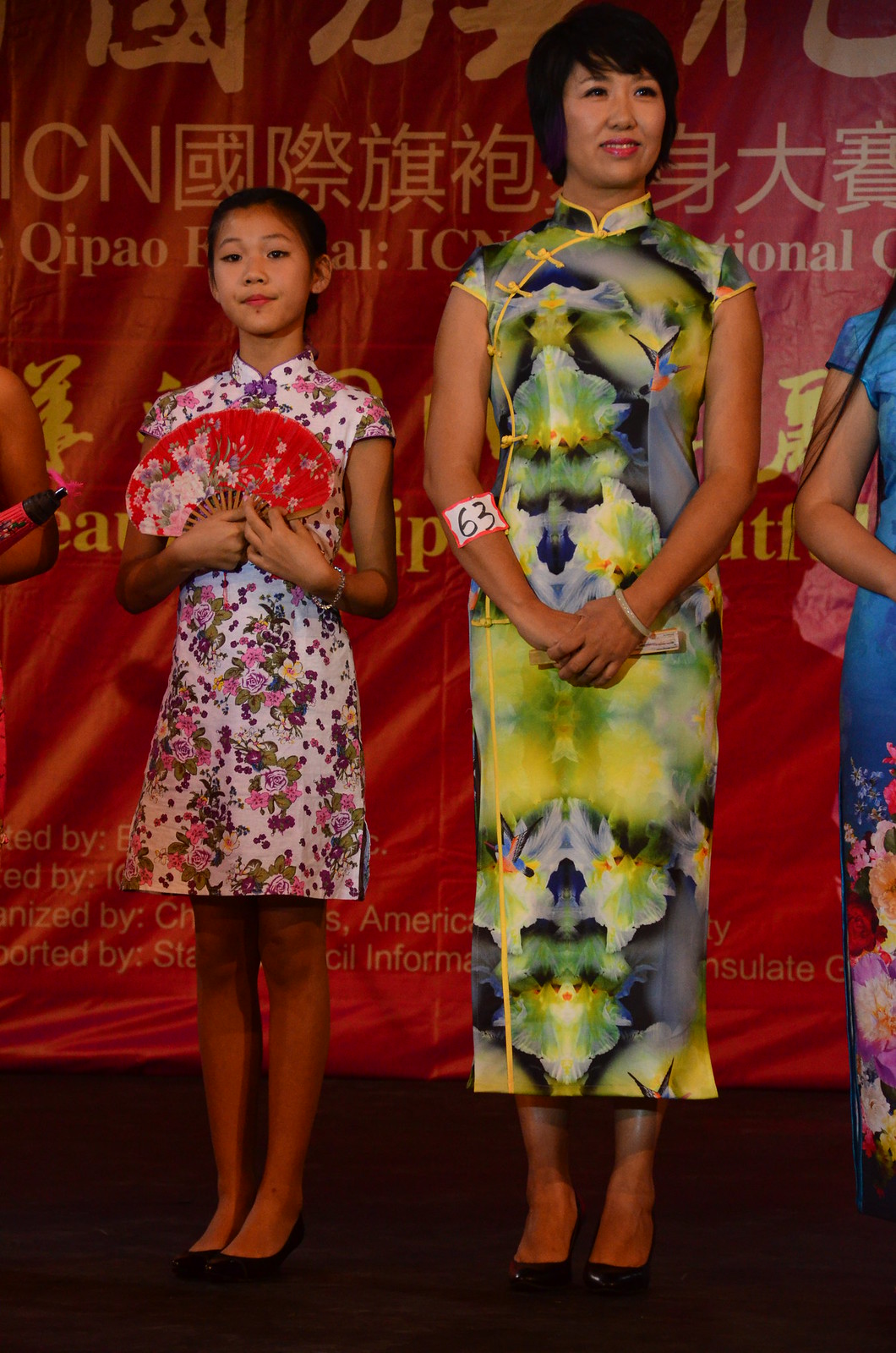This full-color photograph captures a vibrant event in Asia, showcasing an elegantly dressed young girl and a woman, both of Asian descent, standing side by side on stage. The backdrop is a red banner with prominent yellow Chinese characters and partially visible English text, which appears to read "Kuaipao" and "ICN National." The young girl, positioned on the left, is dressed in a charming white floral dress adorned with pinks, purples, and greens, featuring a mandarin collar and short cap sleeves, ending just above her knees. She holds an open red fan decorated with flowers and wears black ballet flats. Beside her, on the right, stands the woman, taller and poised, wearing a multicolored tea-length dress with an abstract print in yellows and blues, also with a mandarin collar and short cap sleeves. A white sticker labeled with the number "63" is affixed to her right forearm. Both individuals are wearing black heels. The photo places them at a well-coordinated event, possibly a beauty contest or a cultural celebration, emphasized by their sophisticated attire and poised demeanor.